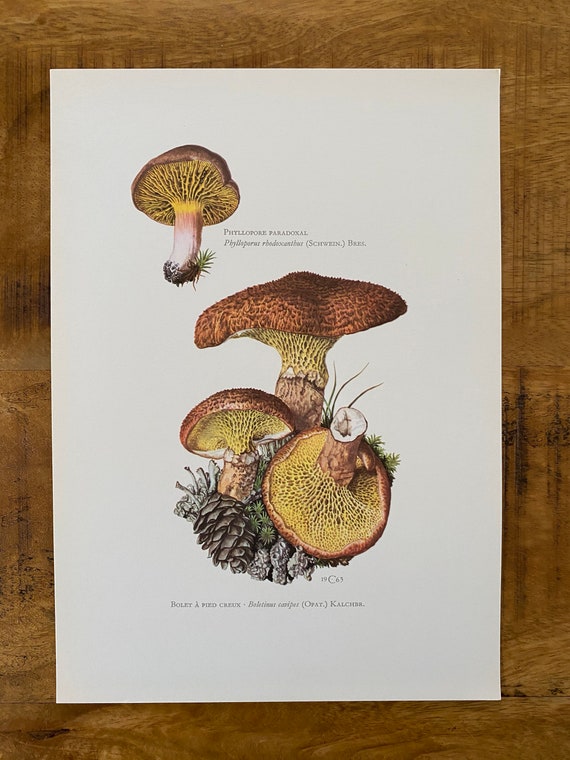This meticulously illustrated portrait depicts a variety of mushrooms, presented on a white sheet of paper with detailed drawings and scientific labels. The artwork, potentially intended for educational purposes, is encased in a thick, rustic wooden frame and lies on a warm, amber-brown wooden table. The primary focus is on the central image featuring three mushrooms, identified as "Bole and Fried Crow." These mushrooms exhibit brown, textured caps with yellowish gills and light brown to white stems. 

In this central cluster, two of the mushrooms remain rooted in the earth, while the third is upturned, revealing its intricate underside. Accompanying this trio, a pine cone and sprigs of greenery accentuate the forest floor setting. Above this group, there is a smaller, single illustration labeled "Fiddlepore Paradoxal" with a small patch of grass at its base.

The mushrooms are vividly detailed, with brown caps and spongy orange-yellow gills. The stems transition from white at the base to light brown towards the cap. Tiny, faint text, presumably the Latin names and other identification notes, accompanies each illustration, although it is largely illegible due to its minuscule size.